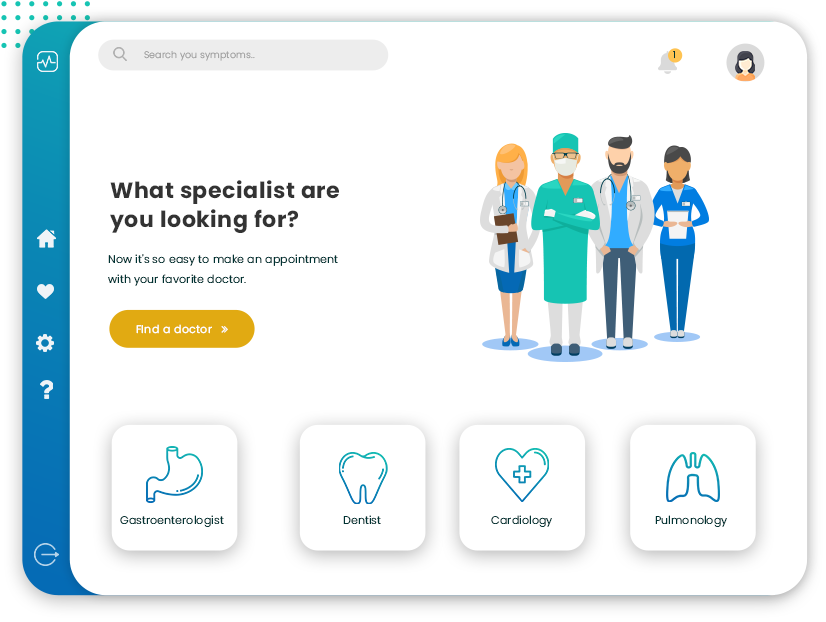The image, seemingly a screenshot from a medical-themed website, showcases a user-friendly interface designed to help patients find and book appointments with healthcare professionals. On the left of the screen, there is a prominent title in black font reading, "What specialist are you looking for?" Just below this title, a brief description explains, "Now it's so easy to make an appointment with your favorite doctor." These elements are followed by a dark yellow button in the center, labeled "Find a Doctor."

To the right of these textual elements, there is a vibrant clip art illustration depicting a diverse group of four medical professionals, including a doctor, a nurse, and two other healthcare providers. Below this visual, the website categorizes medical specialists into four selectable buttons: "Gastroenterologist," "Dentist," "Cardiology," and "Pulmonology."

Additionally, on the left-hand side of the screen, there is a vertical menu with clickable icons for navigation. These icons include a home key, a heart button, a settings gear, and a help icon represented by a question mark.